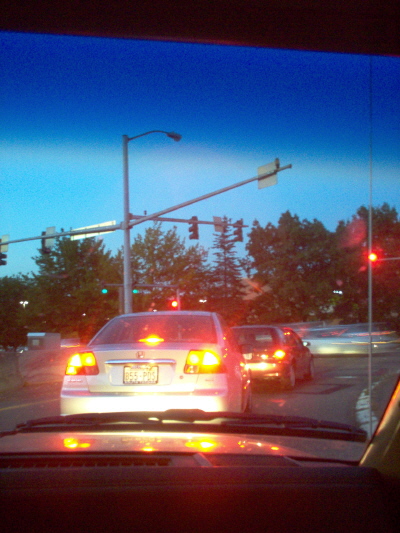This detailed image captures a scene from inside a car, looking through the windshield over the dashboard and past one visible windshield wiper. The photograph, likely taken during early morning or sunset, showcases two cars ahead, both with their taillights on. The nearest car appears to be a silver sedan, and the one in front of it is a reddish small SUV. Both vehicles are stopped at a red traffic light at an intersection. The stoplight is positioned on metal poles to the left and accompanied by additional traffic lights and signs. To the right of the stoplight, there is a curved, white-painted curb. Beyond the intersection, deciduous trees with leaves are visible against a pretty blue skyline. Some blurred movement of other cars with white and red lights indicates light traffic in the distance. The scene suggests the viewer might be a passenger, given the visible frame of the window and absence of a steering wheel.